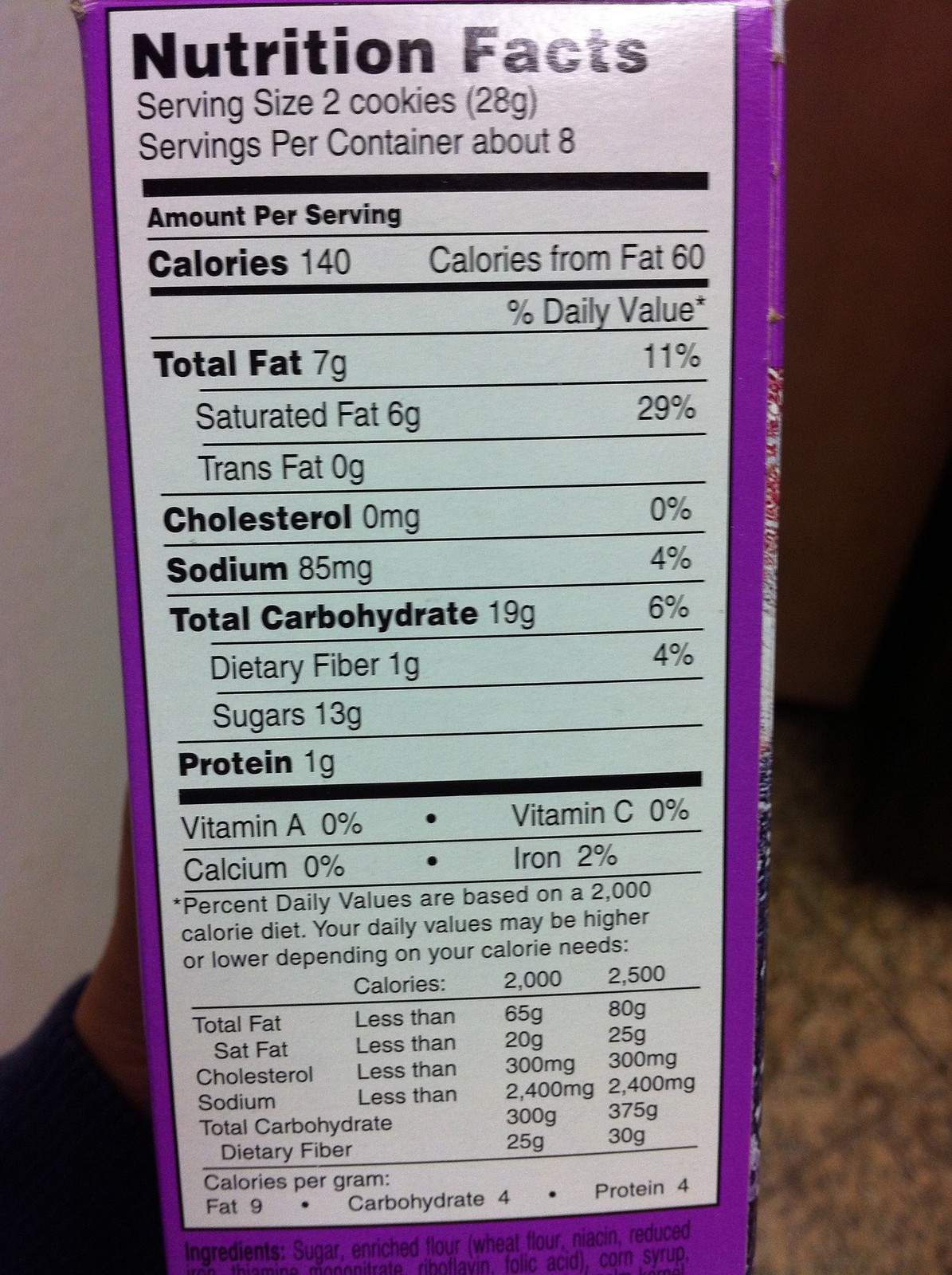The slightly vertical rectangular image prominently features a close-up view of the side of a product box, specifically focusing on the Nutrition Facts label. The background boasts a striking purple border, which frames the inner white section displaying the nutritional information in black lettering. The label indicates a serving size of 2 cookies, suggesting that the box likely contains cookies. In the lower portion of the image, the wrist and lower part of a left thumb are visible, suggesting the box is being held by someone to capture the picture. This hand is clad in a dark-colored sleeve, adding a hint of contrast to the overall color scheme of the image.